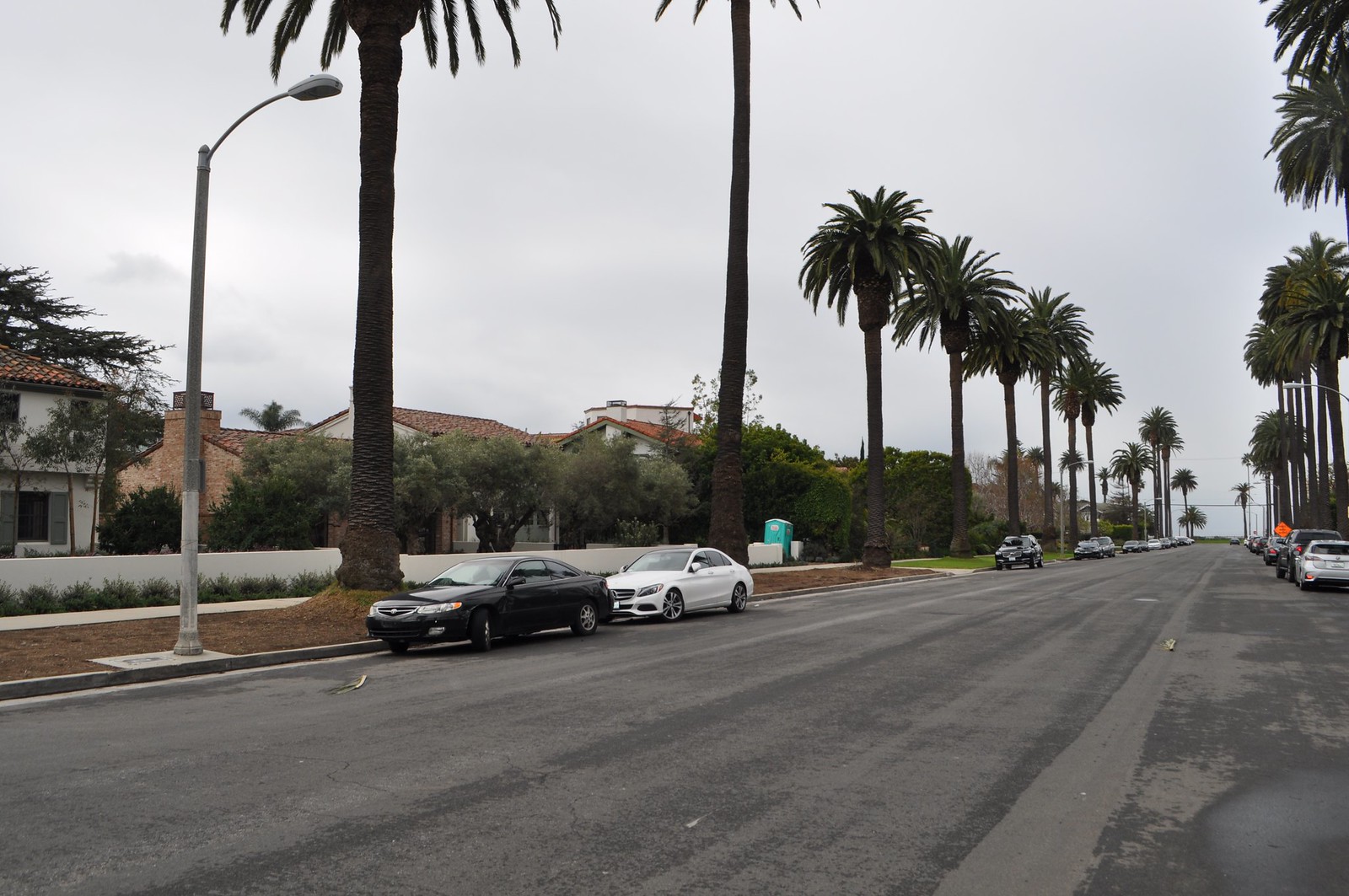A tropical street scene unfurls with towering palm trees lining both sides of an asphalt road that stretches from the bottom left to the middle right of the image. Nestled among the lush greenery, bushes, and various trees, a series of light poles runs down the left side of the street, with a particularly noticeable pole standing prominent. Cars are parked along both sides: a black car and a white car sit closely together on the left, while additional vehicles are scattered further down the road. On the right side, numerous cars span the street, but no buildings are visible. Centrally, behind a wall and partially obscured by some houses with characteristic reddish roofs reminiscent of Florida architecture, stands a humorous sight—a port-a-potty. The sky above is a dull, overcast gray, casting a subdued light over the entire scene, enhancing the tranquil and slightly whimsical atmosphere.